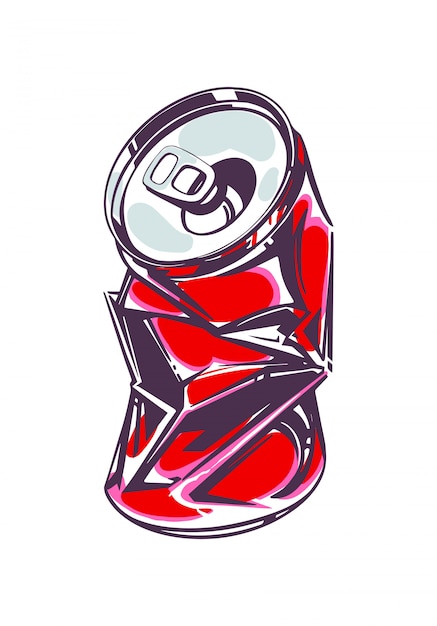The image features a digital, stylized rendering of a partially crushed red soda can against a white background. The can, which appears to be the work of a graffiti artist or cartoonist, stands upright with its base and top remaining mostly intact. The top is silver, slightly bent outward, and the opener has been pulled up, indicating it has been opened. The body of the can is primarily red with white and pink highlights accentuating its crumpled sections, while black shadows provide depth and contrast. Various blotches of purple and dark red add to its artistic, exaggerated style. The crinkles in the can create a dynamic visual, with pink edges surrounding the red circles and solid purple areas in the creased segments, giving it a vibrant, colorful appearance.